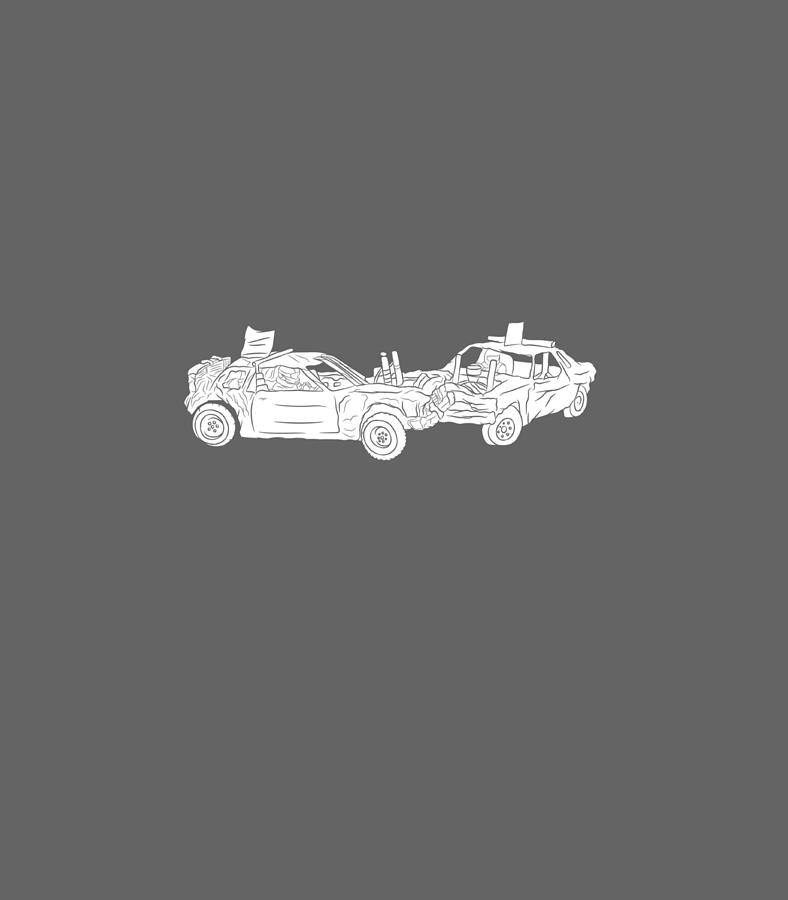This is a simple, monochromatic drawing depicting a head-on collision between two white cars on a dark gray background, with no additional scenery like roads, trees, or buildings. The image is oriented in portrait format and features cars illustrated with black outlines. The car on the left is colliding with its driver's side front fender against the right car's front end. Both vehicles are severely damaged, with crumpled metal, detached panels, and tires in disarray, giving the impression they are racing cars involved in a crash derby. The entire scene conveys a sense of significant impact and destruction at the point of collision.